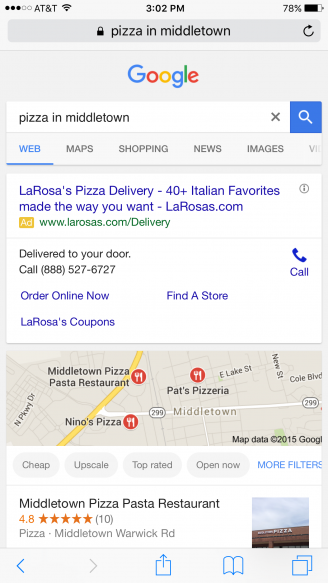A detailed and cleaned-up caption for the image could be:

"This image, captured from the screen of a cell phone, shows a Google search for 'pizza in Middletown.' At the top of the screen, the search options include 'web,' 'maps,' 'shopping,' 'news,' and 'images,' with 'web' selected. The search results highlight La Rosa's Pizza Delivery, featuring over 40 Italian favorites, available at larosas.com. The result emphasizes the convenience of delivery with an option to call or order online, along with a link to La Rosa's Coupons. Below, a map of Middletown displays local pizza places, including Nino's Pizza, Pat's Pizzeria, and Middletown Pizza Pasta Restaurant. A highlighted review indicates that Middletown Pizza Pasta Restaurant has garnered a commendable rating of 4.8 stars from 10 reviews, located on Warwick Road in Middletown."